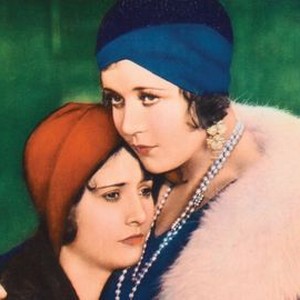The image depicts two women engaged in a sorrowful embrace, their faces visibly marked by sadness. They are adorned in head coverings, with the taller woman on the right wearing a dark blue turban and long pearl necklace, accentuated by earrings. She is dressed in a blue blouse. The shorter woman on the left, who presses her face to the chest of the taller woman, dons a red head covering with some hair poking through and wears black clothing, though the image cuts off, preventing further detail. Set against a fully green background, the emotional connection between them is palpable, reminiscent of the fashion styles of the 1920s, suggesting a low-resolution, vintage photograph or an illustration capturing a poignant moment.